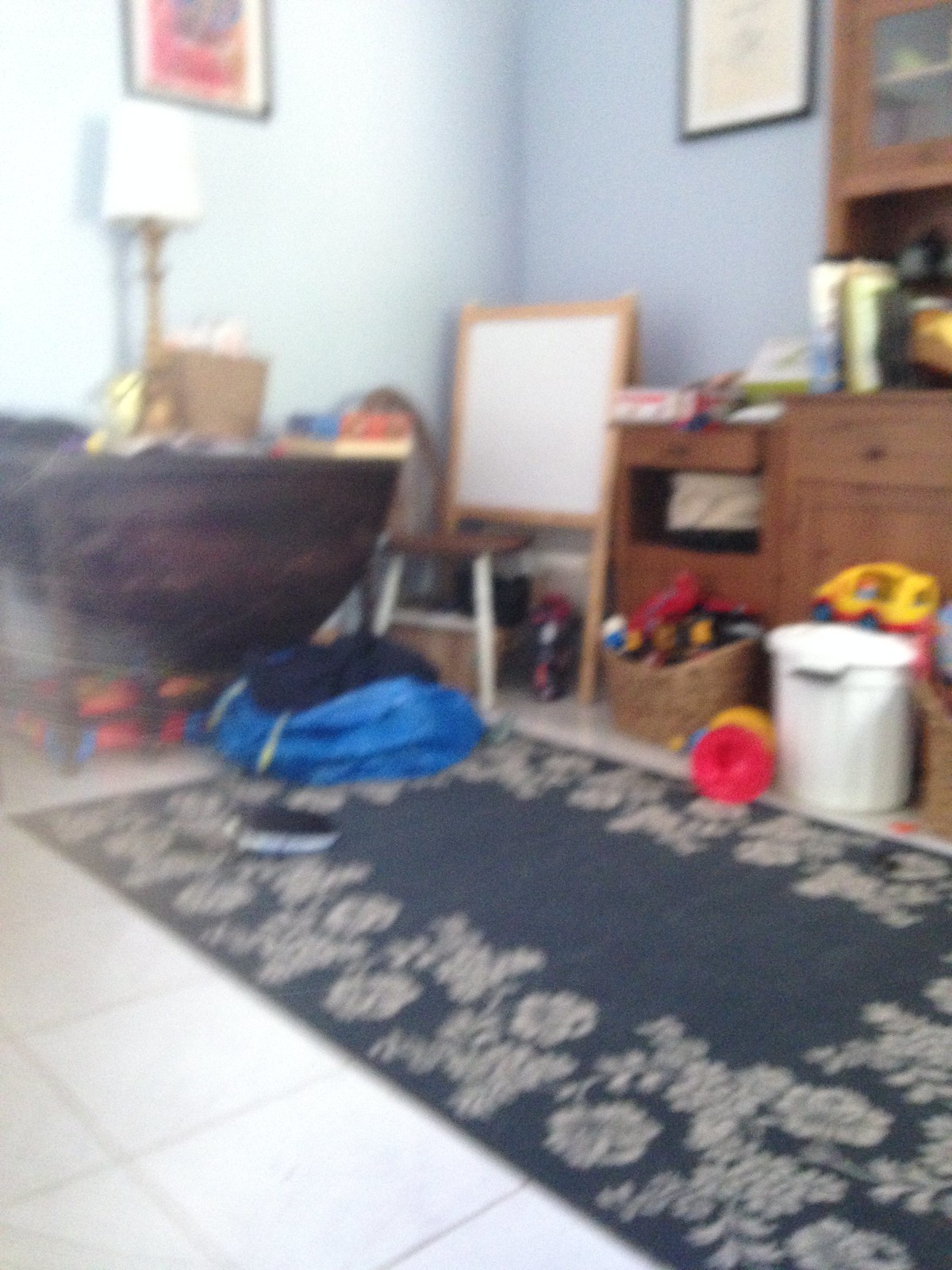A sunlit room, softly illuminated by daytime light, features light blue walls adorned with various pictures. The image, though slightly blurry, appears to be an older photograph likely taken with a low-resolution camera. Central to the room is a brown desk, upon which rests a lamp along with miscellaneous items. In one corner stands a white easel with a whiteboard, alongside a lone chair. A black and white shoe lies casually on the floor, surrounded by an assortment of toys, baskets, and small cars, indicative of a household with young children. Adding to the room's cluttered charm, another shelf and desk brims with various objects, and a garbage can is also visible, contributing to the lived-in feel of the space.